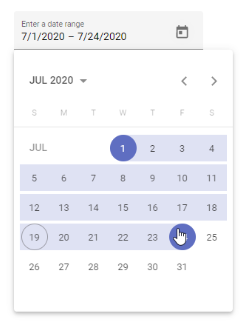The image depicts a digital calendar interface focused on the month of July 2020, set against a plain white background. At the top of the interface, there's a prompt reading "Enter a date range." The user has selected a date range from July 1, 2020, to July 24, 2020. This selection is visually represented on the calendar: July 1st is highlighted with a dark blue circle, indicating the start date, and July 24th is similarly marked with a dark blue circle, signifying the end date. Each day in between, from July 2nd to July 23rd, is filled in light blue, indicating the range duration. Notably, July 19th has a faint circle around it, though it remains uncolored. A finger icon, resembling a pointer, hovers over July 24th, emphasizing the selection's endpoint. The entire calendar is presented without any additional background elements or colors.